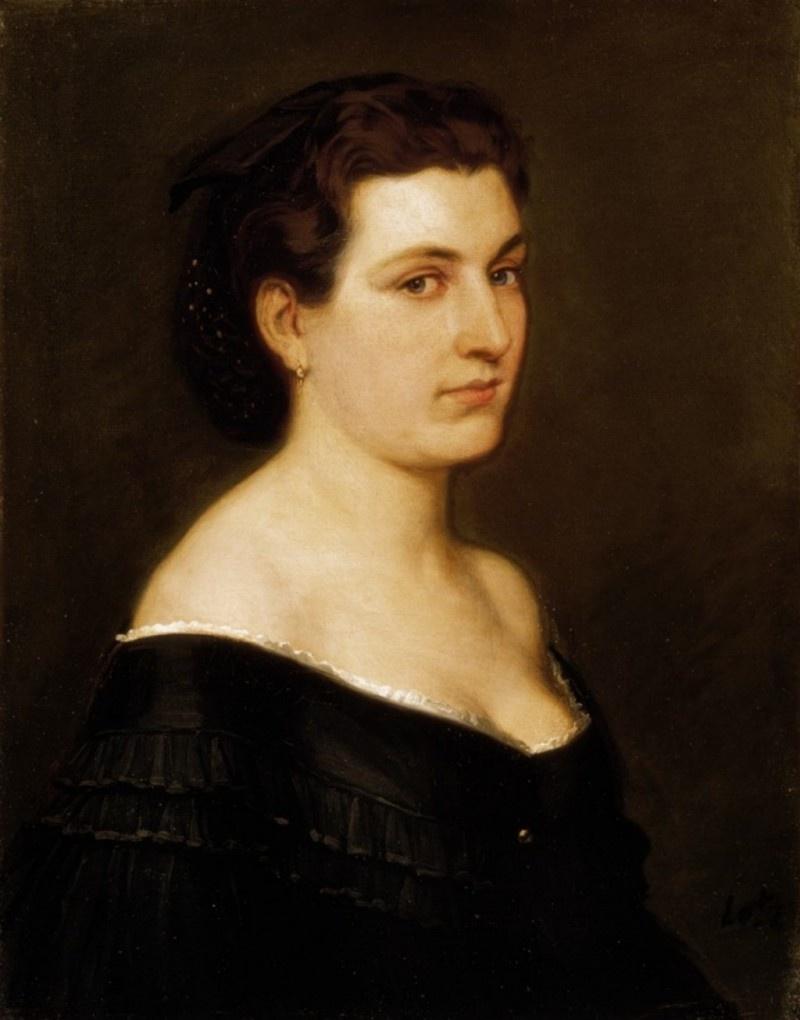The painting depicts a woman centered against a progressively darker brown background, which intensifies towards the bottom of the image. She is wearing an off-the-shoulder black dress adorned with a white frill at the top edge and a single black button. Her light brown hair is styled back with a black cloth featuring white polka dots. She has fair skin and is adorned with a single small gold earring on her right ear. The woman is seated with her body facing right, but her light brown eyes gaze directly forward, giving a sense of direct engagement with the viewer. Her expression is neutral, with closed lips that bear a hint of lipstick. The overall dark tones and classical style of the painting lend it a historical, somewhat medieval, aesthetic.